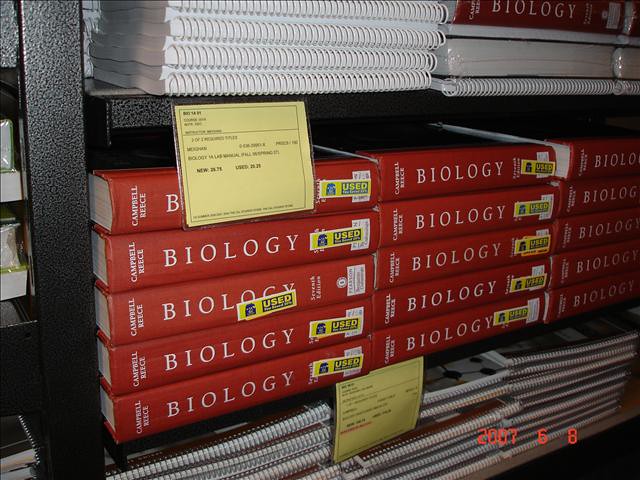The image depicts a black bookshelf with multiple levels, fully stocked with an assortment of biology textbooks and spiral-bound notebooks. On the top shelf, several spiral-bound manuals are visible, while a sideways view of book bindings reveals a red biology book with white text, along with other wire-bound books. The second shelf is dominated by stacks of biology textbooks, with titles by Campbell and Reese clearly visible in white font. Many of these books have yellow and blue stickers indicating they are used. The bottom shelf features a variety of decorated notebooks, including one with a pattern resembling soccer balls. Yellow notes and price tags indicating "new" and "used" status are scattered across the shelves, enhancing the university bookstore vibe. A date in the bottom right corner, "2007-6-8," suggests the image was taken on that day, possibly in a library or student book storage area.